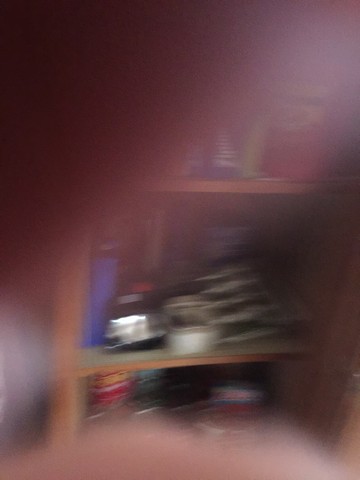A very blurry photograph features a cabinet with two visible shelves. The upper left corner of the image is notably dark, possibly due to an obscuring object resembling an arm. This object transitions from black to a dark grayish-red hue as it stretches across the frame. On the top shelf of the cabinet, slightly to the right, there appears to be a bag of sugar in red packaging next to another indistinct bag. The middle shelf holds a tall, blue bottle on the left, which might be a drink, a roll of silver duct tape in the center, and a black and silver item placed horizontally whose nature is unclear. At the bottom, various items rest, though they are indiscernible due to the extreme blurriness of the photograph.